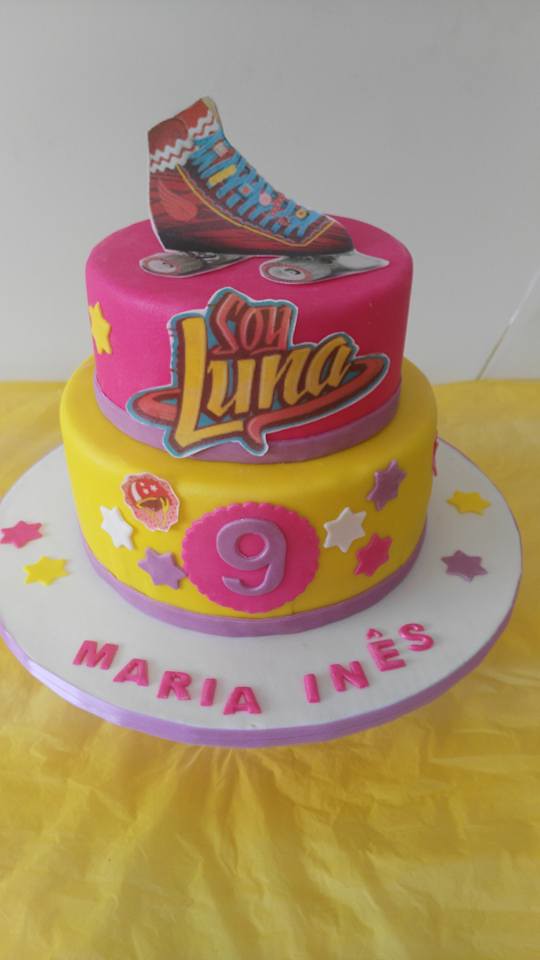This vibrant birthday cake, designed for a child, features two tiers and is set against a white background. The cake rests on a white platter with a lavender trim, laid out on a yellow tablecloth, possibly made of paper or crepe. The lower tier is covered in yellow fondant, adorned with a lavender number 9 and complemented by fondant stars in pink and yellow tones. The upper tier is hot pink, topped with a paper cut-out of a roller skate for a playful touch. The base of the cake platter proudly displays the name "Maria Inez" in pink capital fondant letters. The overall theme, highlighted with the inscription "Soy Luna" on the top tier, indicates a colorful and joyous celebration for a nine-year-old girl.